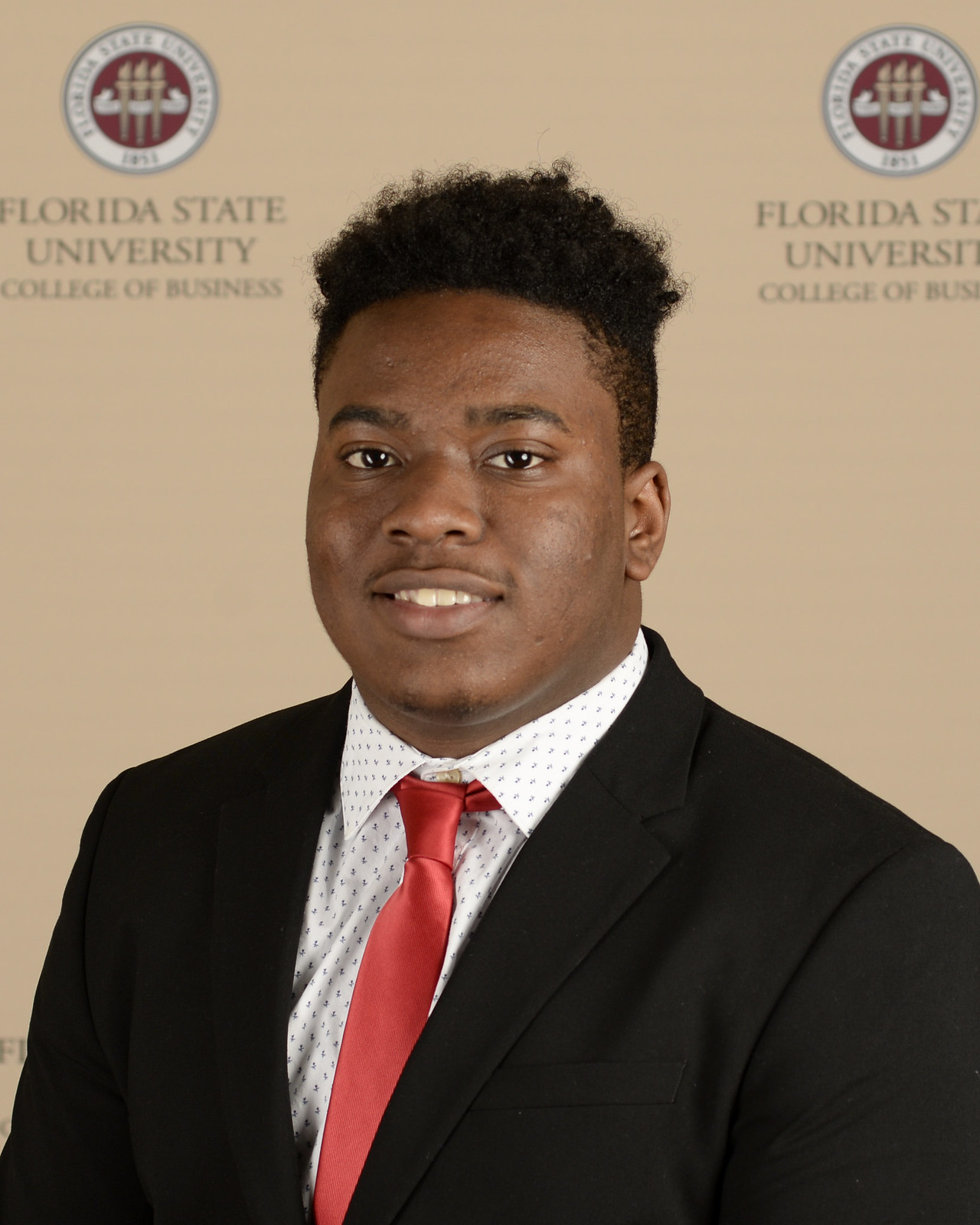This is a detailed, color photograph of a young African American man, likely college-aged, taken indoors. He is seated and facing the camera with a slight smile on his rather round face. His short black hair is styled in a fade, cut low on the sides and higher on the top. He is dressed in a professional black suit with a narrow lapel, a white dress shirt adorned with a small pattern of gold or brown markings, and a shiny pale red tie that is slightly loose around his neck. The backdrop is a very light tan wall with the Florida State University College of Business logo and seal printed twice, flanking his head on either side. The logo appears to include the year 1851. The overall setting and attire suggest that this could be a formal portrait likely intended for a yearbook or a college-related publication.